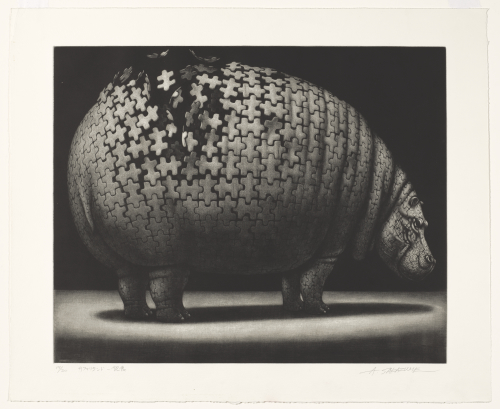The image features a highly detailed, monochromatic artistic representation of a large hippopotamus, constructed from interlocking jigsaw puzzle pieces. Set against a solid black background, the hippopotamus stands out distinctly due to its light gray, puzzle-piece-patterned skin. The animal, facing to the right, is depicted with short legs and a large, distended belly, emphasizing its massive size. Notably, the puzzle pieces on its back appear to be disassembling, creating an impression of movement and fragmentation. This disarray in the puzzle pieces extends upwards, adding a dynamic element to the composition. A white ring around the bottom of the hippopotamus suggests its shadow, with a black spot in the middle enhancing the depth. The entire image is framed by a white border, within which, on the lower right corner, faint initials “A-N-S” are inscribed, hinting at the artist’s signature.